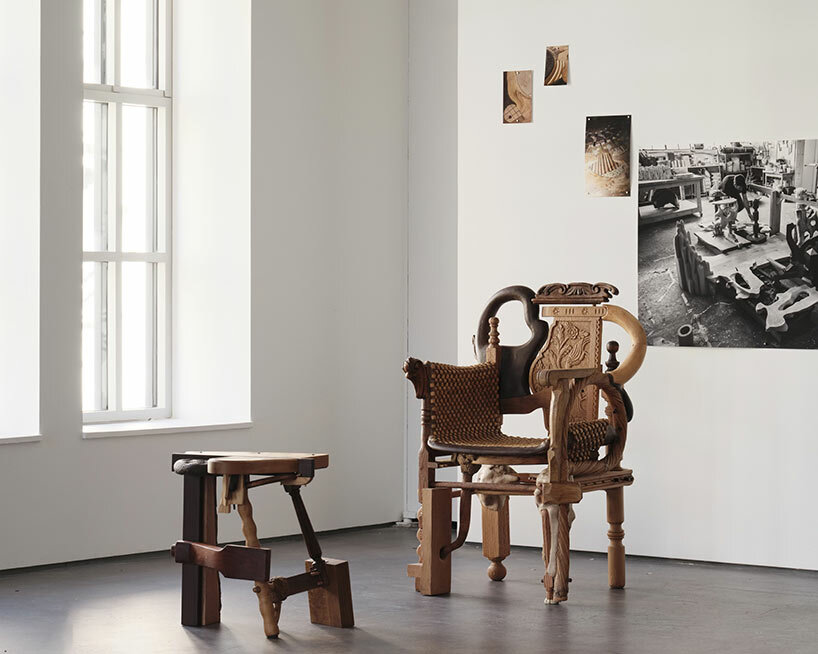The image depicts a minimalist room with white walls and a dark-colored floor, featuring a large, ornately designed wooden chair placed centrally. The chair, composed of both light and dark wood, stands out due to its unique and eclectic structure. Each of its four legs is distinct: one has a rectangular portion ending in an orb, another is a dowel with central etchings, the third is a multi-colored twisted piece, and the fourth is a rectangular block with a hole halfway down. The chair's back showcases various cutout shapes, including a heart-like design, crafted from two different woods. The armrests also differ; one has a straight out design with a curved end and a circular support underneath, while the other appears to have an animal head carving. A beaded surface runs from the right armrest under the seat. 

In front of the chair is a small footstool made of mismatched wooden pieces, echoing the chair's diverse design. Hanging on the white wall behind the chair are four photographs, three smaller ones and a larger black-and-white one, seemingly of a carpenter in his workshop. These images appear to document the chair's construction process and add a narrative element to the room's minimalist aesthetic. Additionally, there is a bright white light streaming in from the left side windows, suggesting a sunny day outside.